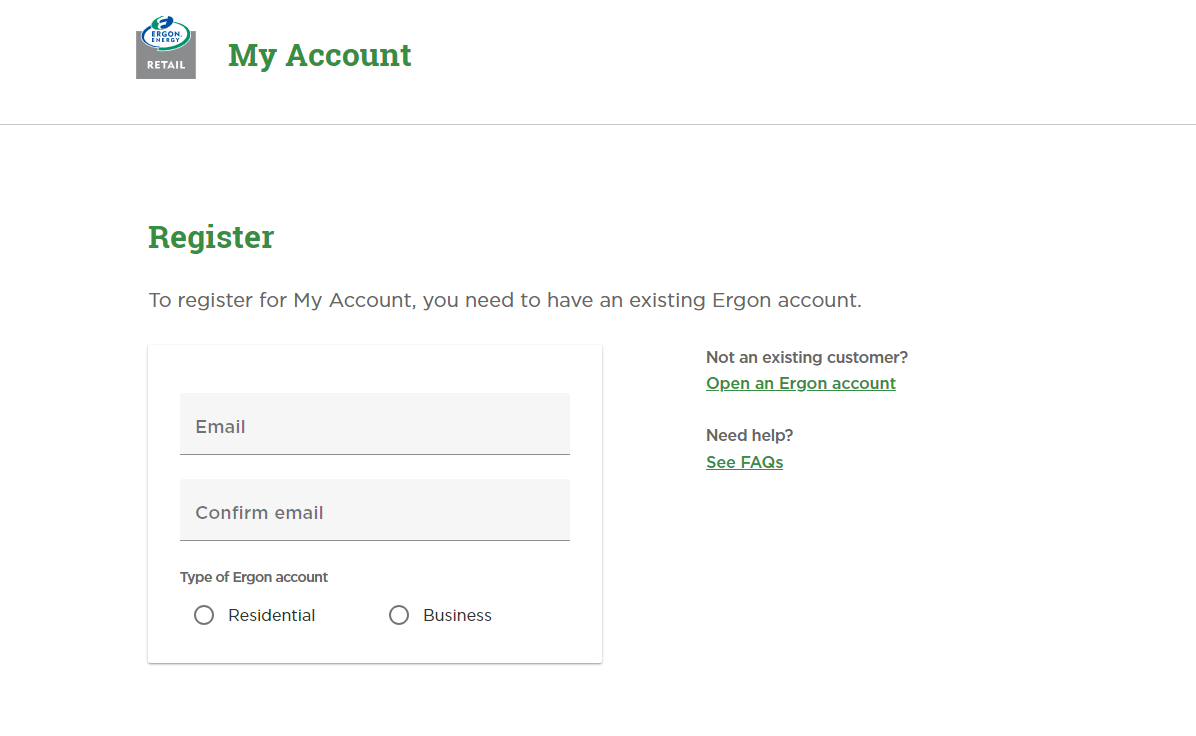The image depicts a webpage interface for Ergon Energy's account registration feature. At the top, there is a small gray square with the word "RETAIL" written in white, capital letters. Adjacent to it, on the right, there is a circle outlined in blue and green with the words "Ergon Energy" inside it. Next to the circle, the text "My Account" appears in green font. Below this, a thin gray line separates the header from the rest of the content.

Directly beneath the line, the word "Register" starts with a capital 'R' and is displayed in green letters. The subtext indicates that to register for a "My Account" with Ergon Energy, an existing Ergon account is required, with "My Account" and "Ergon" emphasized through capitalization of the letters M, A, and E.

Further down, there is a form area with fields for "Email" and "Confirm Email." Below these fields, there are two selectable options for the type of Ergon account, labeled with circles for "Residential" and "Business."

Outside of this form, a message in green text reads, "Not an existing customer? Open an Ergon account." Additionally, another green text box states, "Need help? See FAQs," providing links or additional guidance for users.